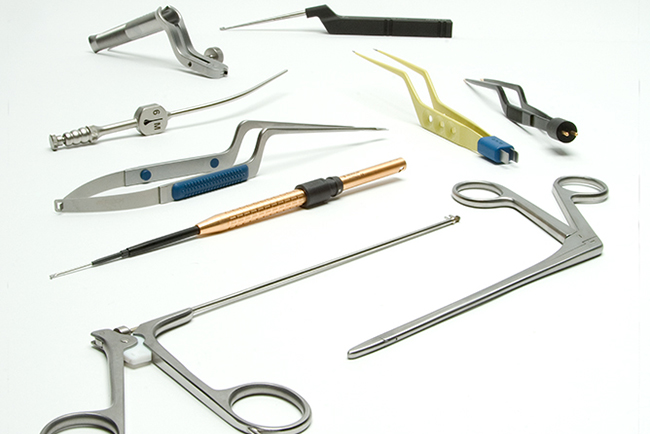The image displays a collection of nine precision tools meticulously arranged on a light greenish-gray background that gradates to white in the lower right corner. The tools are predominantly metallic, featuring a palette of silver, gold, and brass, ensuring their potential for easy sanitization. Among the instruments are many exceptionally sharp tweezers and clamps, alongside a variety of specialized pliers often used in surgical or mechanical assemblies.

On the top left, there is a silver tool with a unique gun-like shape. To its right, in the top central position, sits a long, flat silver object with a black handle and a sharp, pointed tip. Other notable instruments include a needle encased in gold with a black handle, and two more distinct tweezers: one gold-colored with a blue band that is longer, and another shorter, silver version with a black band. Highlighted also is a long, angled tool with a gold base and a silver point, encased in black.

Additionally, the assortment includes needle-nose pliers with various colored handles—one entirely metallic with blue on the handle, another yellow with blue details, and one in black. The layout also showcases two peculiar scissor-like tools positioned sideways at a 90-degree angle, indicating their specialized usage. All these tools sit meticulously on a white table, each designed for high precision in accessing small, intricate areas.